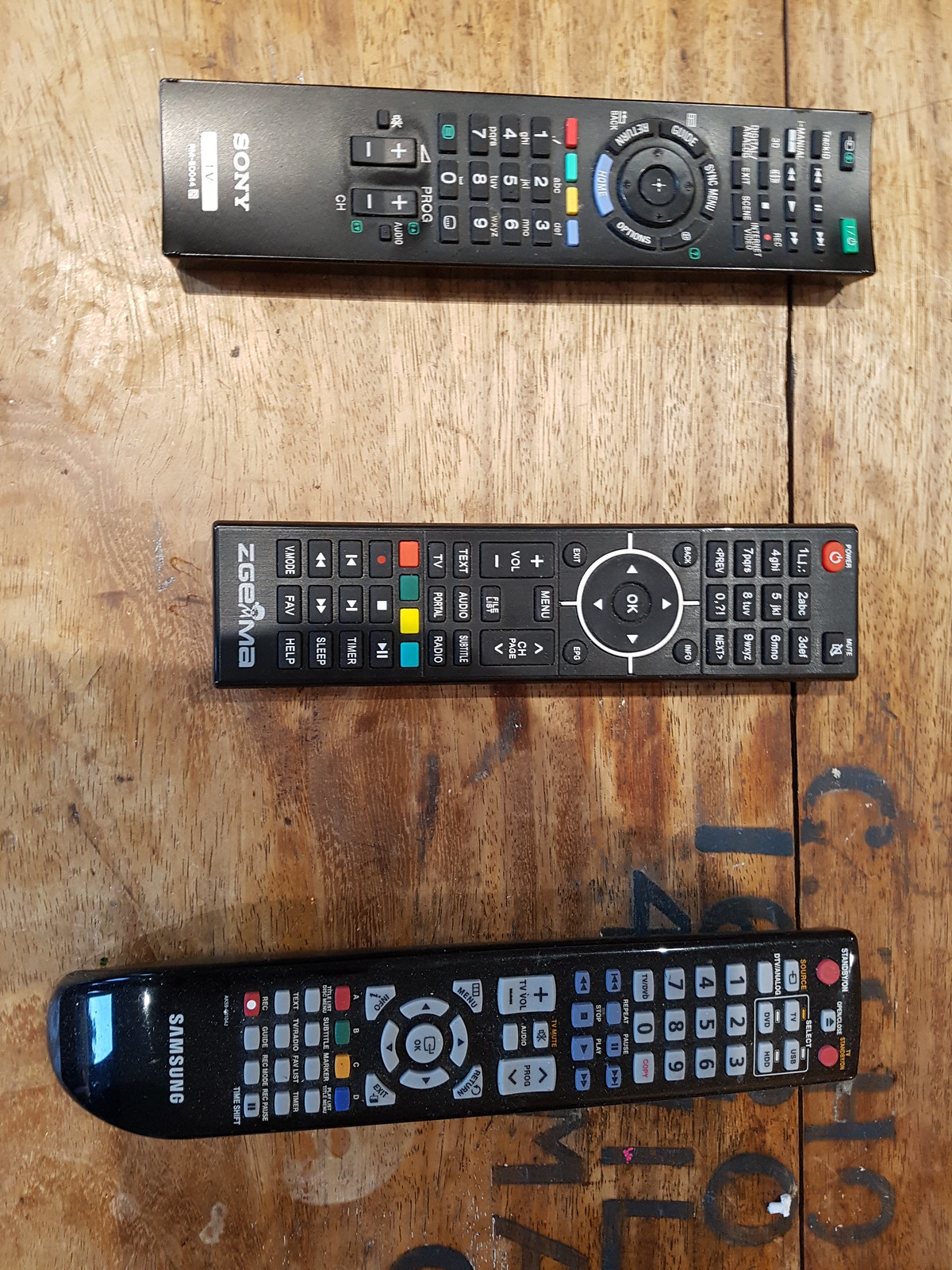In the image, three TV remote controls are neatly arranged horizontally against a brown wooden desk, viewed from above. The wooden desk features a slot with hinges, suggesting a liftable section, though it is currently closed. The remotes, facing to the right-hand side, vary slightly in size and design. The topmost remote is a Sony, with predominantly black buttons and a distinctive row of red, green, yellow, and blue buttons. In the middle lies a slightly smaller ZGE AMA remote, also featuring mostly black buttons. The bottom remote, a Samsung, is the longest, characterized by light gray buttons and notable red dots on the right-hand side which serve as the power buttons. All remotes are black, and their varying button colors and brands highlight their distinct designs and functions.